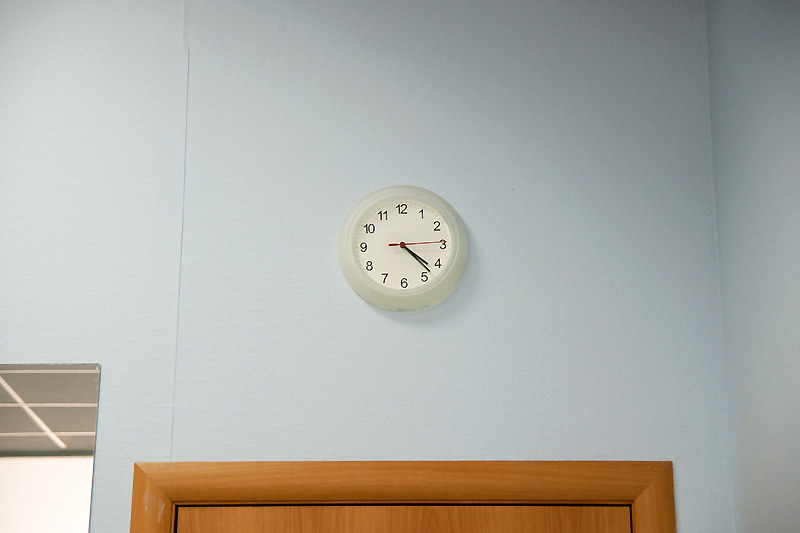This detailed photograph depicts a room with light blue-grey walls and a central focus on a round clock positioned above a dark brown wood-framed door. The clock, housed in an off-white circular frame, features a white face with black numbers and black hour and minute hands. The red second hand is nearing the three, while the hour and minute hands are between four and five. The door beneath the clock reflects light, although its source is unseen. To the left of the door, there seems to be either an open doorway or a mirror reflecting another room, revealing a white wall and tiled ceiling with white grout. A thin strip along the wall suggests a division, possibly due to wallpaper or a fold. At the bottom left, a slight peek of what appears to be a mirror edge is visible, and the wall's corner extends out towards the viewer on the right side of the image.